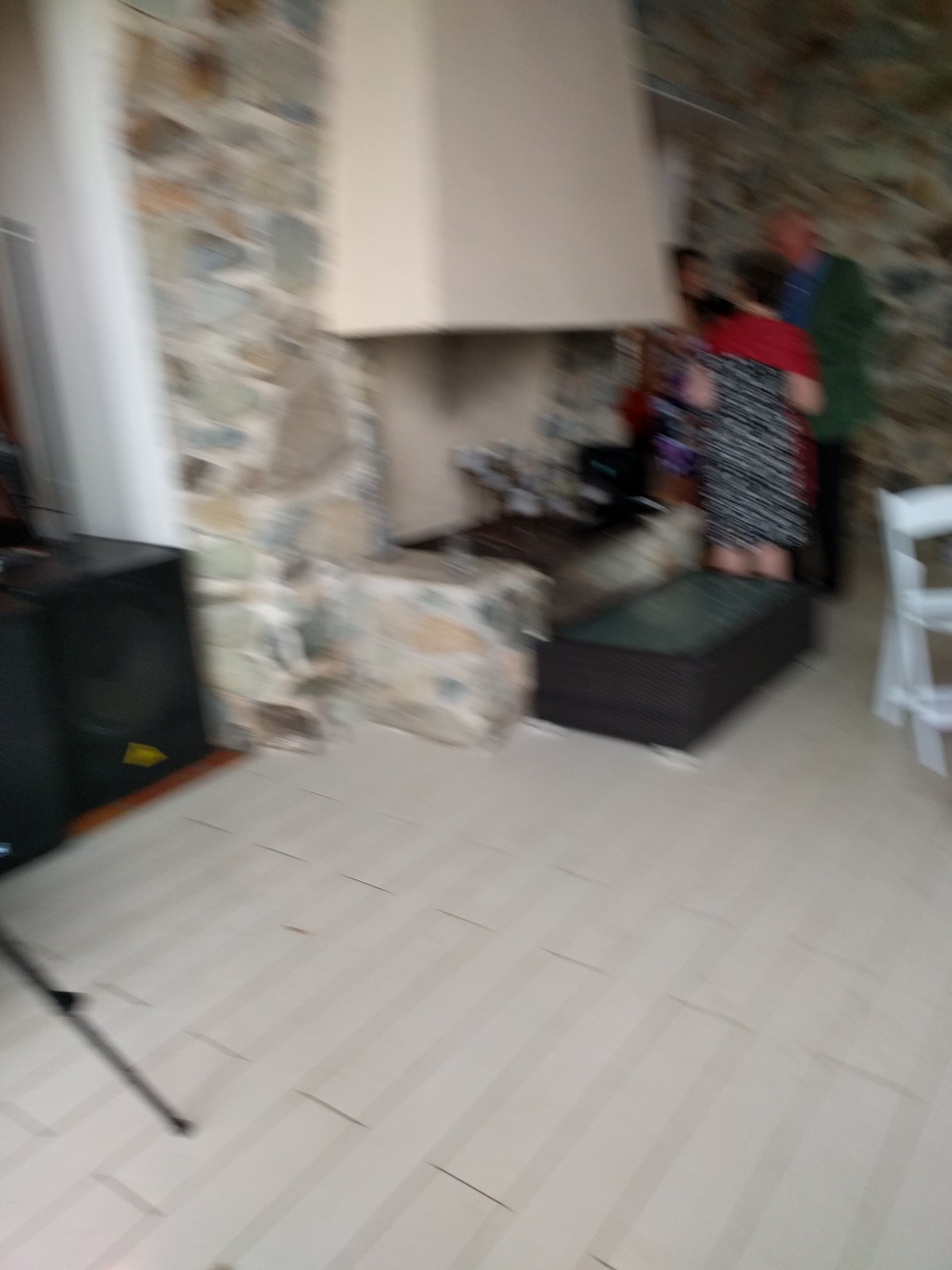This blurred indoor photograph depicts three people engaged in conversation in a corner of a room. The group includes an older gentleman in a green sweater layered over a blue shirt, and two ladies—one in a black and white dress with a red shawl, and the other whose details are less clear. They stand against a wall composed of various colored stones, giving it a bedrock or stone tile appearance. On the right side, there's a distinctive white wooden chair resembling a ladder, and beside it, a walking cane with a rubber end can be seen on the white wooden planked floor. Above the lady in the black and white dress is a cream-colored canopy, and behind her, a stand is visible. Additionally, to the left, there are two black speakers situated near a fireplace with a white covering.